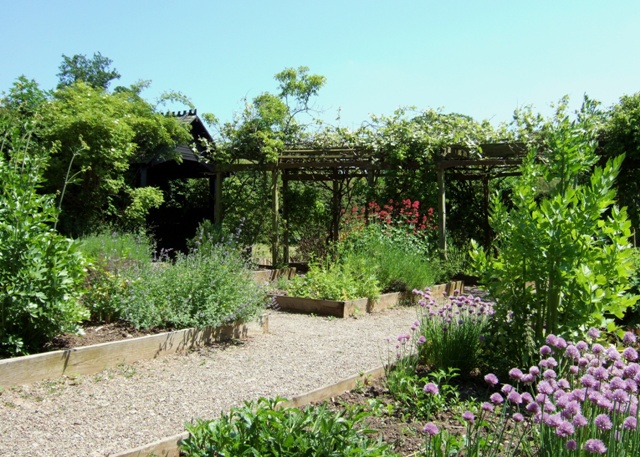This image features a considerable-sized, picturesque backyard garden or courtyard bustling with vibrant flora. A diagonal gravel pathway, bordered by unstained light wooden 2x4s, gently guides the eye through the garden starting from the bottom left and meandering toward the back right. Elegant trellises and beams extend across the path, providing support for hanging plants and creating a canopy of greenery. On the right side of the foreground, tall green leafy plants and stunning orchid-colored flowers stand out prominently. The garden boasts a rich variety of green shrubs, larger bushes, and trees that form a lush backdrop, while pops of color from red, white, and pink flowers enhance its charm. Towards the center and bottom right, there are clusters of vibrant blooms. In the distance, partially obscured by verdant foliage, a roof structure—possibly a gazebo or a small house—emerges into view, with the clear blue sky visible beyond, lending an inviting atmosphere to the scene. Scattered gnomes populated amongst the flowers add an almost whimsical touch, completing this serene and beautifully detailed landscape.